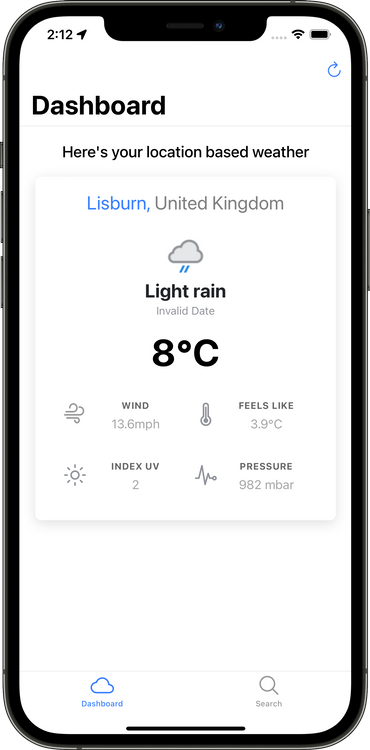This image is a cell phone screenshot displaying a weather dashboard. The screenshot captures the black outer edge and the side buttons of the phone. The background of the screen is a very light gray.

In the upper left-hand corner, bold black text indicates the time, accompanied by a send arrow icon. On the upper right, icons for Wi-Fi, battery status, and four gray dots in a row are visible. Approximately two lines down on the right edge, there is a blue reload button.

On the left side, two lines below the Wi-Fi and battery icons, bold black text reads "Dashboard." A light gray horizontal line separates this from the weather information below.

Centered under the horizontal line, the dashboard displays a weather section titled "Here's your location-based weather." The location is highlighted in a white square at the top, with "Lisburn" in blue text and "United Kingdom" in gray text beneath it. Below this, a gray cloud icon with blue rain signifies rain.

Clearly centered and in bold black text, the weather condition is labeled "Light Rain." Directly under this description, in very small light gray letters, the text "Invalid date" appears.

Further down, in bold black letters, the temperature is given as "8°C." About three lines beneath this on the left side, a wind icon is present with the word "Wind" next to it, followed by "13.6 MPH."

To the right of the wind information is a thermometer icon. Next to this, it reads "Feels like 3.9°C." 

A few lines down, a sun icon is displayed with "Index UV" beneath it, followed by the value "2." Next, a heartbeat graph line icon indicates the atmospheric pressure, with "Pressure" next to it and "98.2 mbar" below.

At the bottom of the screen, there are two functional buttons labeled "Dashboard" and "Search."